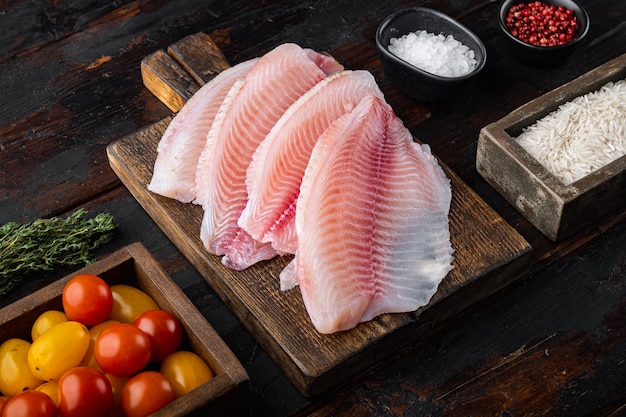This is a meticulously arranged food photo taken from a rightward angle above a dark, weathered wooden table. On the left side of the table, a rustic wooden square box brims with vibrant yellow and red cherry tomatoes. Positioned in front of the tomatoes are sprigs of fresh rosemary. Centrally placed on the table is a sturdy wooden paddle cutting board with its handle oriented towards the top left. The board showcases four uncooked, pink-hued fish fillets, potentially salmon, meticulously laid out side by side, revealing the rich muscle texture of the fish. Adjacent to the right of the cutting board is a smaller rectangular wooden box filled with dry white rice. Above this box, a little black circular container holds sea salt, while another identical container, placed to the right, is filled, possibly with cranberries or peppercorns, adding a touch of contrast to the scene. The composition is carefully balanced, highlighting the fresh and raw ingredients in a harmonious culinary display.